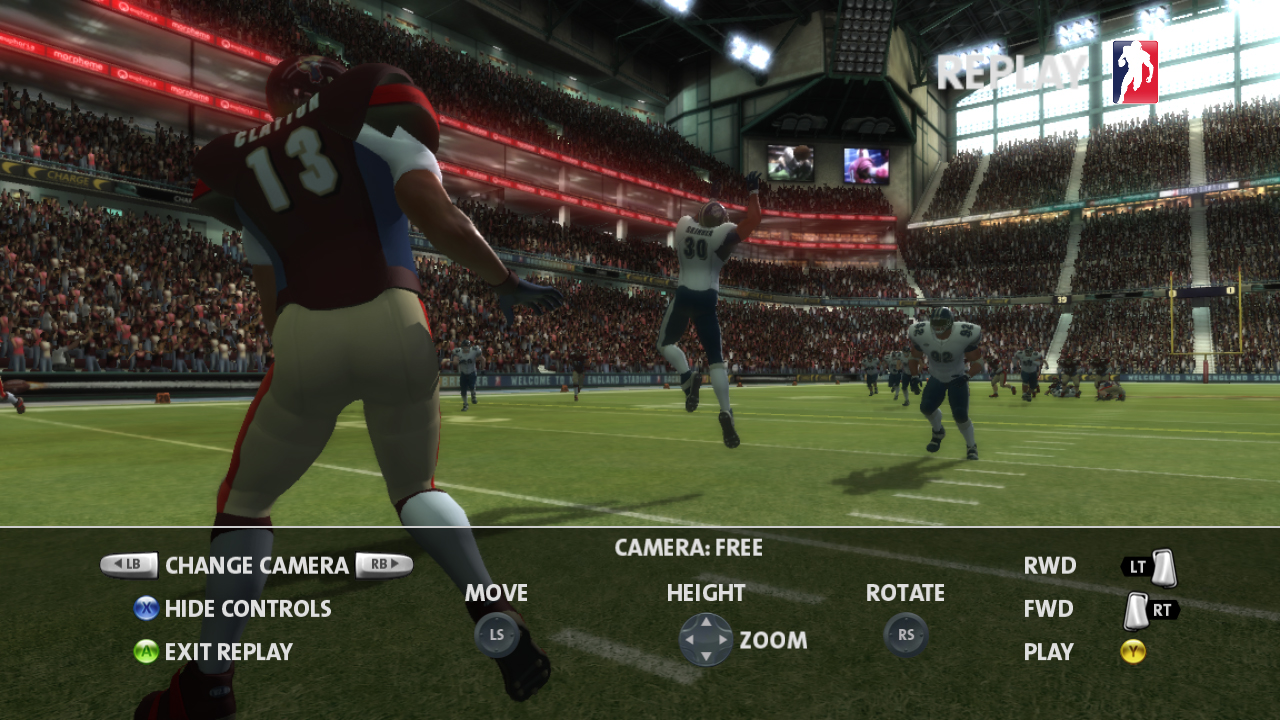The image is a detailed screenshot from a football video game, capturing a replay moment. In the top right corner, the word "Replay" is prominently displayed. At the bottom of the screen, various control options are listed, including "Change Camera," "Hide Controls," "Exit Replay," "Camera Free," "Move," "Height," "Zoom," "Rotate," "RWD," "FWD," and "Play," along with the corresponding button mappings.

The scene takes place on a vibrant green football field marked with white lines. At the center of the action is a player wearing jersey number 13, appearing to have just thrown a football. Surrounding him are other players in white and blue uniforms, engaged in the game. In the background, the stadium's seating is packed with spectators, adding to the atmosphere of a lively sports event.